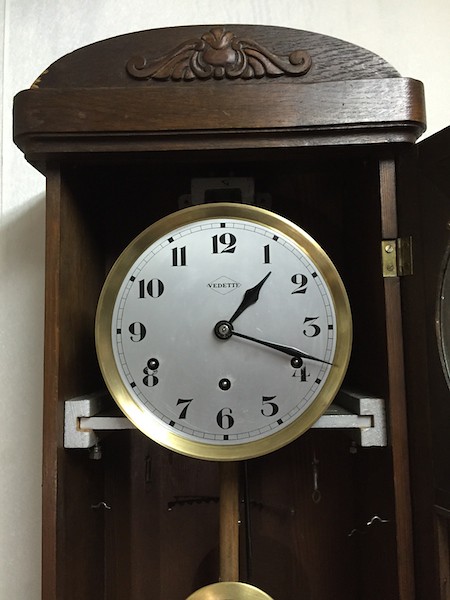The image showcases an ornate grandfather clock housed in a tall, dark wooden cabinet, almost black in appearance. The clock is framed with a brass trim and features traditional numerals from 1 to 12, eschewing Roman numerals. The time displayed is approximately 1:18, with the shorter hour hand just past the "1" and the longer minute hand hovering slightly above the "4." The cabinet door, which is open to reveal the clock face, has gold hardware along its right side. A visible gold pendulum hangs beneath the clock face, indicating its mechanical nature. The design includes a decorative scalloped piece at the top, reminiscent of a miniature London telephone box. The brand name "Vedette" is inscribed in a sideways diamond shape on the clock face, and the natural light in the room casts a shadow on the clock, highlighting its intricate details.